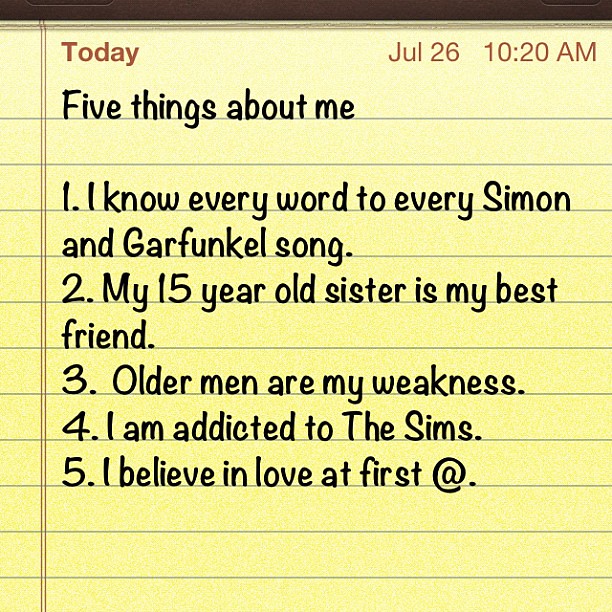The image depicts a color illustration of a square-format, lined yellow notepad. At the top, there's a black horizontal strip resembling a spine. On the left under the strip, "Today" is written in a reddish text, while on the top right, the date "July 26" and the time "10:20 a.m." are noted. Below this header, in modern curved black script, the title "Five Things About Me" introduces a numbered list. Each entry in the list is written in black text: "1. I know every word to every Simon and Garfunkel song. 2. My 15-year-old sister is my best friend. 3. Older men are my weakness. 4. I am addicted to The Sims. 5. I believe in love at first @." The background maintains the classic yellow lined paper look, with the lines and text meticulously aligned. Additionally, thin, reddish-brown vertical lines frame the list on the left side of the notepad.